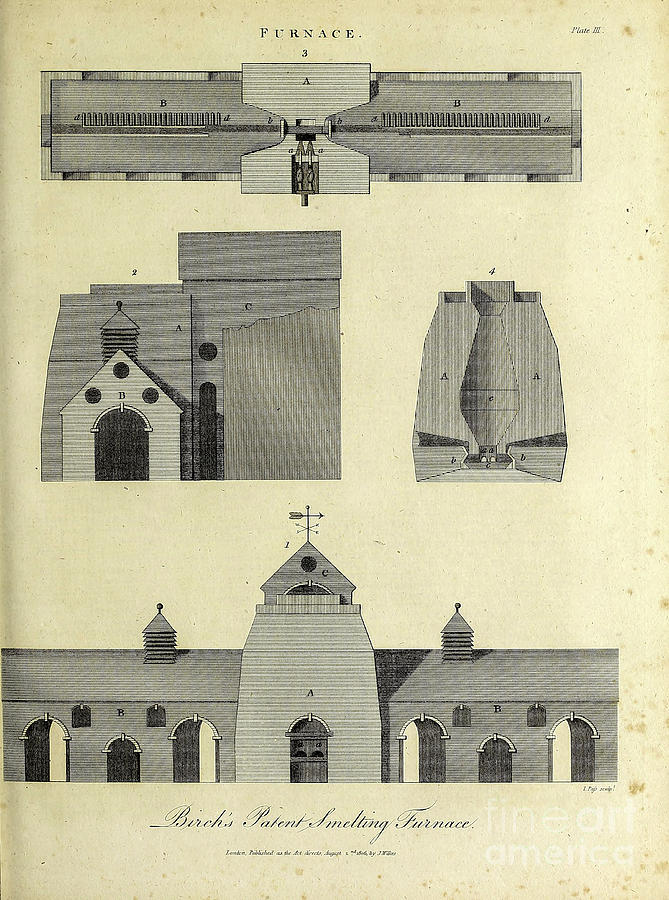This image is a detailed, line-drawn sketch of Birch's patent smelting furnace, featuring multiple views and schematic details. At the bottom of the image, there is a front view of the building, showcasing seven arched doors and a weather vane atop the structure. Above this, two images depict sections of the schematic in the same meticulous line art style, though the specific parts are not easily identifiable. The uppermost section of the image showcases an indoor cross-section labeled A and B, providing insight into the interior layout of the building. Numbered labels and some sparse text, including the words "furnace" and “Birch’s patent smelting furnace," annotate the diagram, offering additional context. The entire sketch, seemingly hand-drawn with pencil, displays a vintage quality, emphasized by stains on the paper. The drawing is displayed flat and oriented towards the viewer for clear visibility of the four distinct sections—top, side, front views, and an indoor cross-section—highlighting both the architectural elements and intricate details of the smelting furnace design.